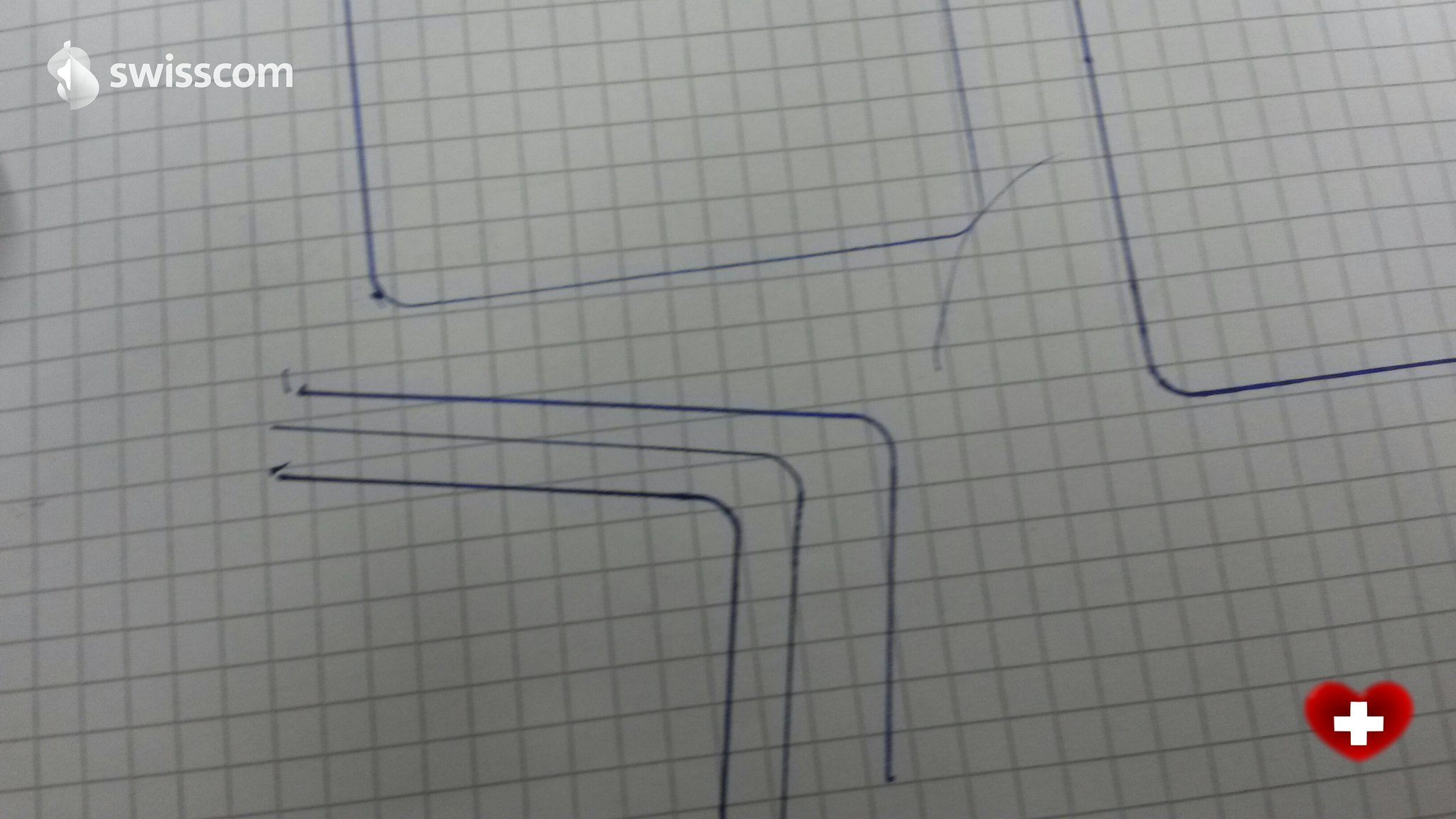This photograph captures a piece of grid paper adorned with various drawings and markings. In the upper left-hand corner, a logo and the word "Swisscom" are prominently displayed in white, uppercase letters. In the bottom right-hand corner, there is a red heart with a white cross centrally positioned within it, reminiscent of the Swiss flag.

The grid paper features a quarter-inch by quarter-inch grid pattern. Pen lines are evident on the paper, suggesting that someone was sketching or outlining shapes, possibly boxes. Two distinct outlines appear to depict boxes, while three additional lines resemble sideways L-shapes. These drawings utilize different instruments: one in black ink, one in what appears to be pencil, and another in blue ink.

Interestingly, smudges mark the starting points of the blue and black ink lines, while the pencil lines remain clear. These smudges are also present in the larger sketches, providing clues about the beginning and end of each drawing process. The juxtaposition of clear and smudged lines adds character to the paper, making one ponder the creative process behind these markings.